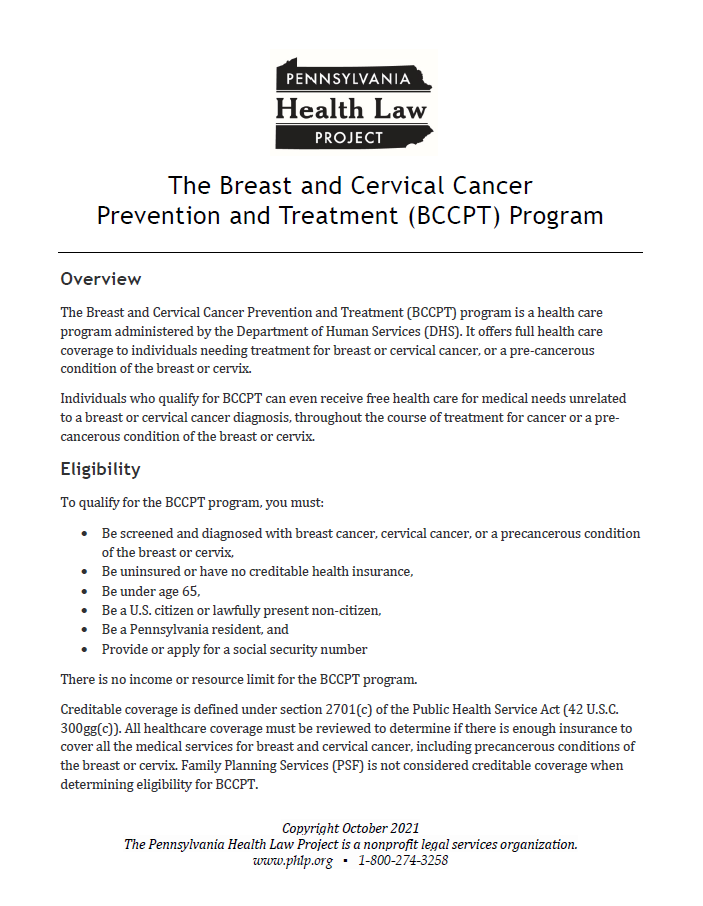This image is a screenshot of a document from the Pennsylvania Health Law Project. The organization's logo features a stylized depiction of the state of Pennsylvania in black, white, and blue colors. The document is titled "The Breast and Cervical Cancer Prevention and Treatment (BCCPT) Program." 

The overview details that the BCCPT Program is managed by the Department of Human Services (DHS) and provides comprehensive healthcare coverage for individuals diagnosed with breast or cervical cancer or a precancerous condition related to these cancers. These individuals can receive free healthcare for all medical needs during the course of their treatment. 

To be eligible for the BCCPT Program, one must meet the following criteria:
- Be screened and diagnosed with either breast cancer, cervical cancer, or a related precancerous condition.
- Be uninsured or lack credible health insurance.
- Be below the age of 65.
- Be a U.S. citizen or a lawfully present non-citizen.
- Reside in Pennsylvania.
- Provide or apply for a social security number.

The program has no income or resource limit. The document concludes with legal disclaimers and a copyright notice dated October 2021.